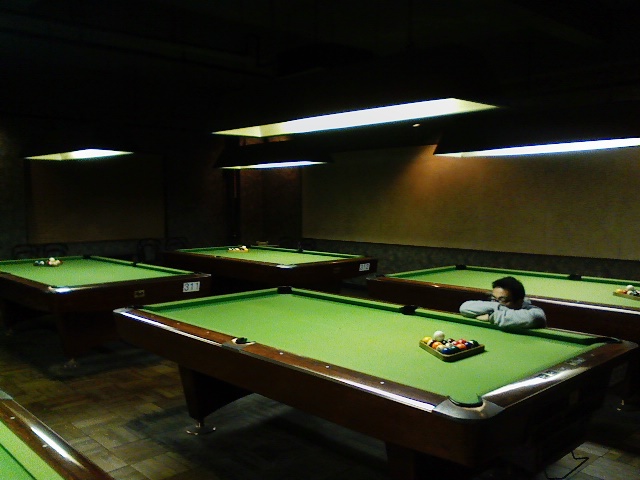The photograph showcases an expansive, dimly-lit pool hall with dark wooden walls and a parquet floor. The room contains four prominently featured billiards tables, each with a bright green playing surface and a brown wooden frame. The tables are evenly illuminated by overhead light fixtures suspended from the ceiling, casting a stark contrast against the otherwise shadowy ambiance of the space. Each billiards table has a neatly arranged triangle of colorful balls, ready for a game. In the bottom right corner of the image, a man with short dark hair, wearing a long-sleeved shirt, is seen crouching on one of the pool tables. He has his arms folded over the table and is intently examining the arrangement of balls, seemingly contemplating his next move. The layout of the room extends from the bottom right to the middle, with a partially obscured fifth table peeking from the left corner, enhancing the depth and spaciousness of the scene.